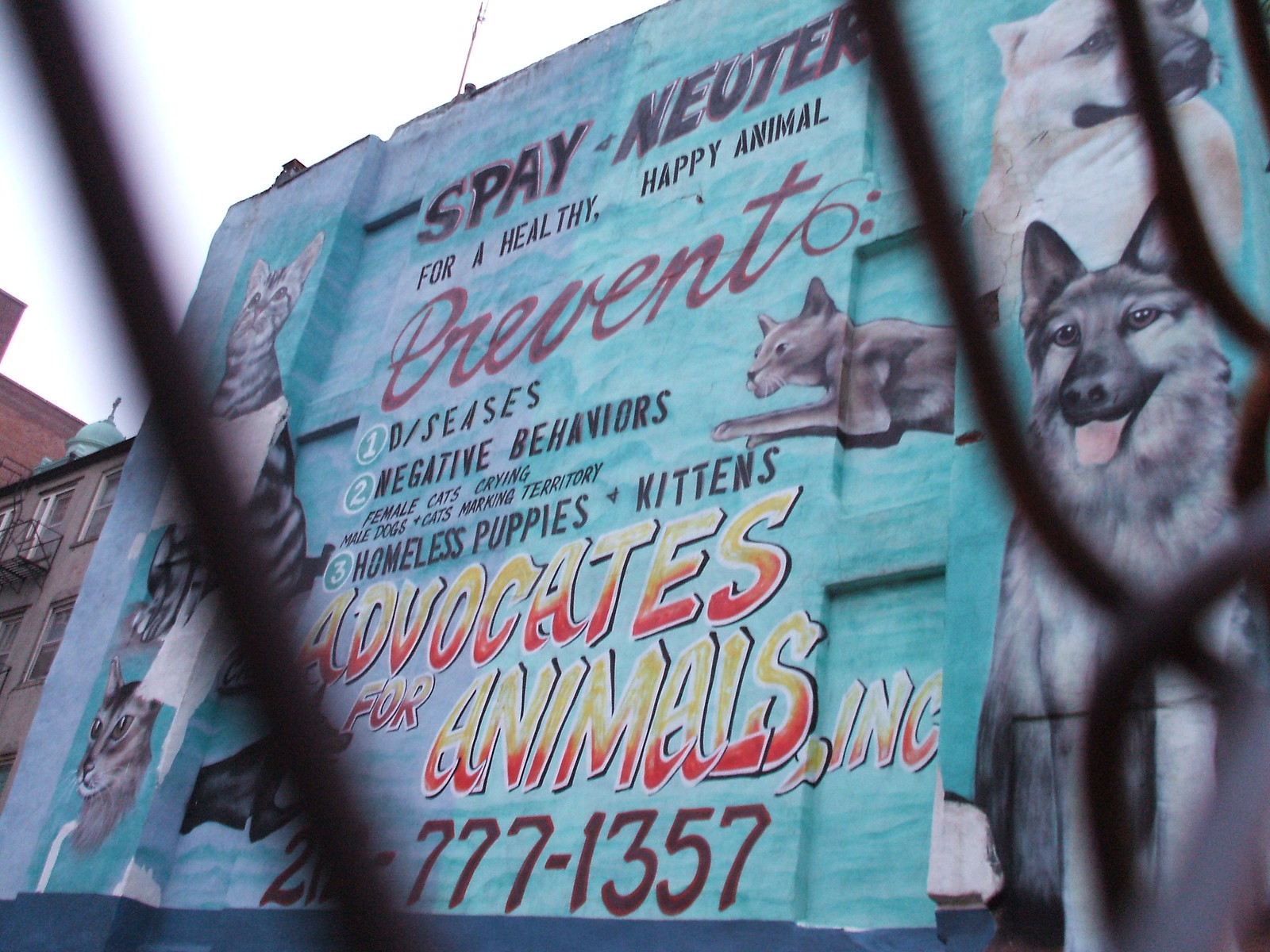The advertisement is a mural painted on the side of a building, featuring a vibrant teal aquamarine background. The focal point is a series of texts and images rendered with a spray-paint aesthetic. The central, prominent black text with a red border reads, "Spay-Neuter for a Healthy, Happy Animal." Below this, in red, it lists benefits such as preventing diseases, negative behaviors, homeless puppies and kittens, with specific mentions of preventing female cats crying and male dogs and cats marking territory. At the bottom, the text "Advocates for Animals, Inc." is stylized in striking yellow and red. The mural is framed by various illustrations of animals, including a notable German Shepherd in the front corner and several cats scattered on both the left and the right sides. Part of the image is taken through a chain-link fence, which partially obscures some of the text. There's also a phone number provided, though only part of it is clear: 777-1357. The mural, with its colorful and lively depiction, dominates the visual space, creating a compelling and informative outdoor advertisement.